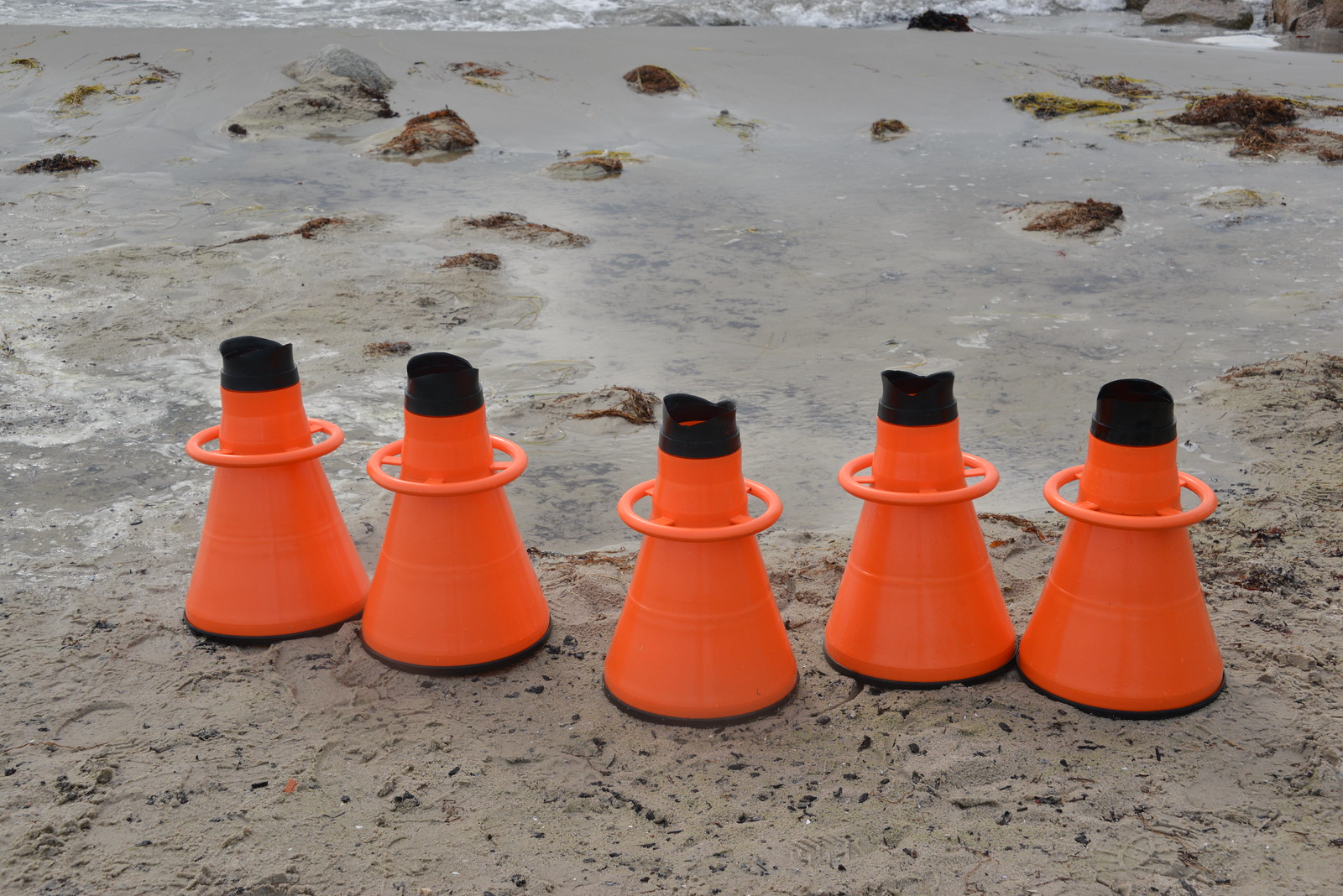In this photograph of a beach, the foreground prominently features five orange buoys with broad, rounded bottoms tapering into skinnier tops capped in black. Each buoy is equipped with a handle, presumably for easy carrying or securing. The beach itself is characterized by a mix of brown sand and rocky patches, with a considerable amount of seaweed washed ashore. Towards the top of the image, the waves break gently along the coast. The scene captures the serene yet rugged beauty of the shoreline and its functional maritime elements.